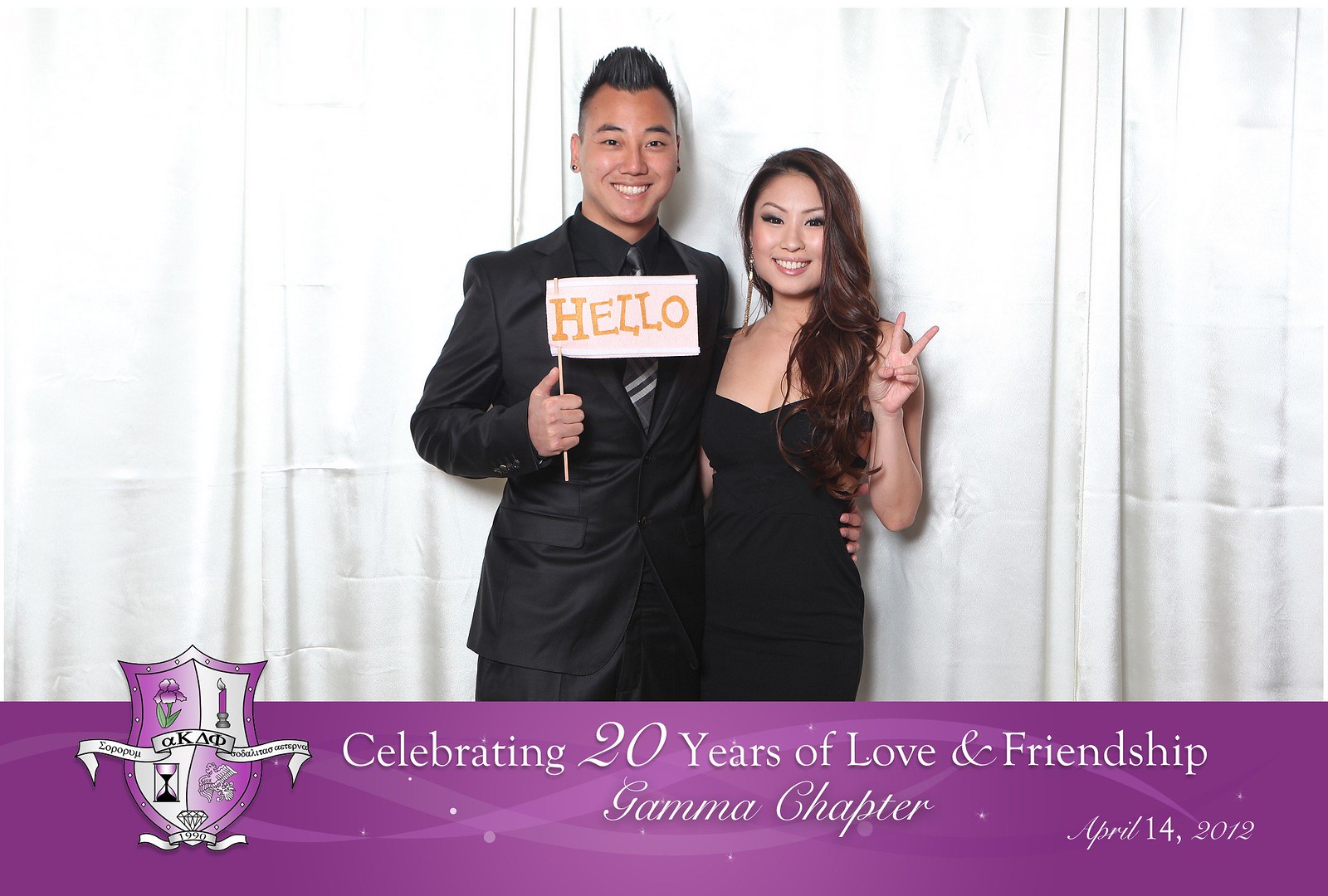The image captures a well-dressed couple posing in front of an elegant white curtain backdrop. The man sports a black suit with a black stripe tie, while the woman stuns in a black evening dress. Both share striking dark hair. The man is holding a small sign that reads "Hello," and the woman playfully flashes a peace sign, possibly denoting their 20-year milestone. At the bottom of the image, a purple rectangle occupies the lower fourth, featuring a shield-like emblem adorned with a rose, a candle, a timepiece, a bird, and a diamond. The white text on this strip reads, "Celebrating 20 Years of Love and Friendship, Gamma Chapter, April 14, 2012."